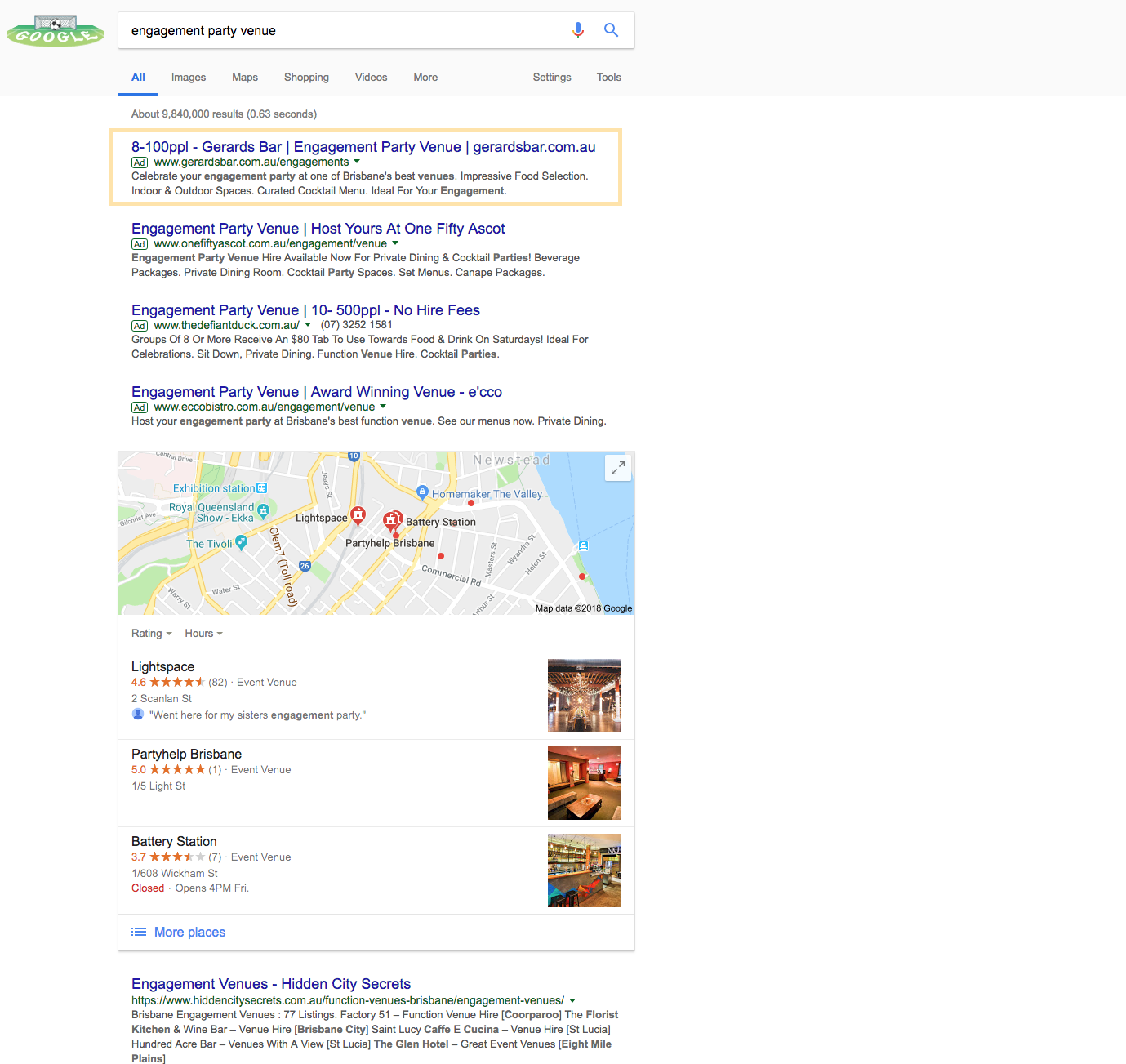The image depicts a search results page with a search bar at the top where the query "engagement party venue" has been entered. The first result is highlighted by a tan-colored rectangular box. It reads: "100 PPL Gerard Bar engagement party venue" with the URL gerardbar.com.au beneath it. Below this, there is a partially legible description mentioning, "Celebrate your engagement party at one of Brisbane's best venues with an impressive food selection. Indoor and outdoor spaces are available," though some of the text is blurry and difficult to read. The second result features the text: "Engagement party venue - host yours at 150..." followed by an incomplete statement. It suggests hosting an engagement party for a range of 10 to 500 people without any hire fees. Further down, it mentions an "award-winning venue" for engagement parties.